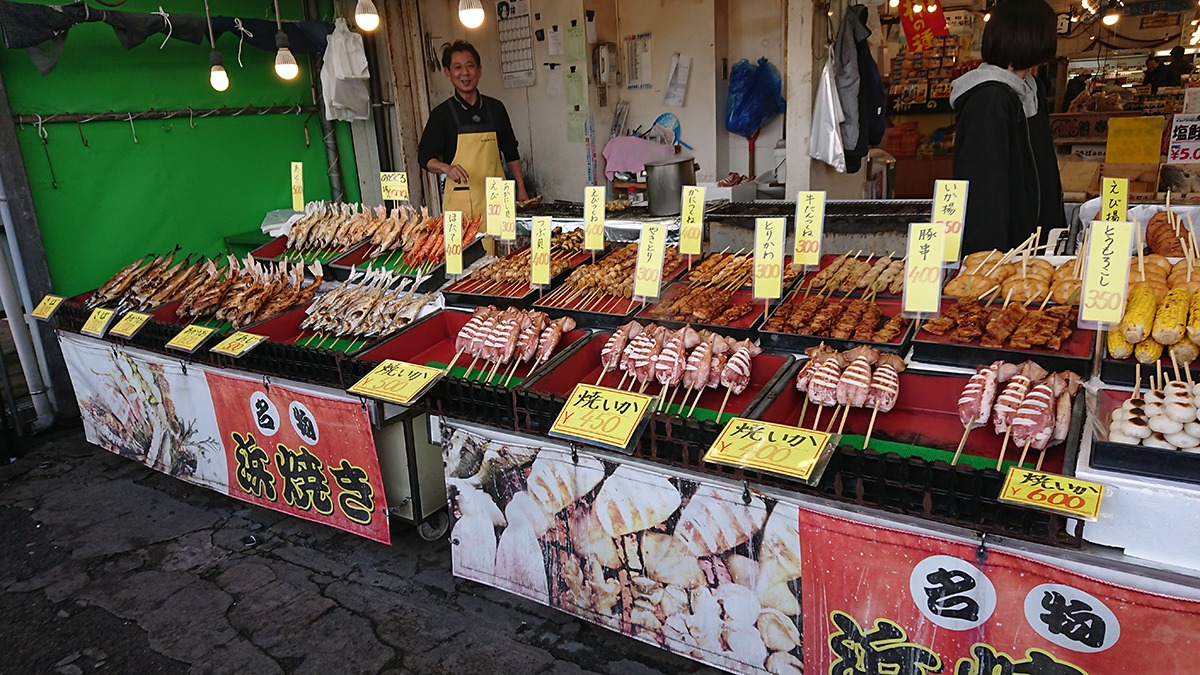The image captures a vibrant food stand at an outdoor market, likely in an Asian country, with detailed characteristics suggesting it might be in Japan. Central to the scene is a smiling man, presumably the vendor, donned in a yellow apron over a navy collared shirt. He stands behind an extensive display of food items arranged neatly in eight columns and three rows, featuring a variety of meats on skewers, including fish, chicken, pork, and beef. Complementing these are non-meat options such as corn on the cob, fried fish, shrimp, crusted bread, and potentially rice cakes. 

The stall itself is adorned with two posters showing pictures of fish, each accompanied by circular symbols and Asian lettering at the bottom, hinting at Japanese writing. The prices of the items range from 300 to 600 yen, indicating a diverse selection tailored to different preferences and budgets. Adjacent to the vendor, another individual, possibly an assistant, is partially visible, seemingly engaged with other customers. The scene is bustling with activity, typified by a concrete floor that extends into the market from the foreground, embodying the lively nature of this open-air market. The backdrop, cluttered with personal items like a calendar, enhances the authenticity and everyday charm of this vibrant culinary setting.